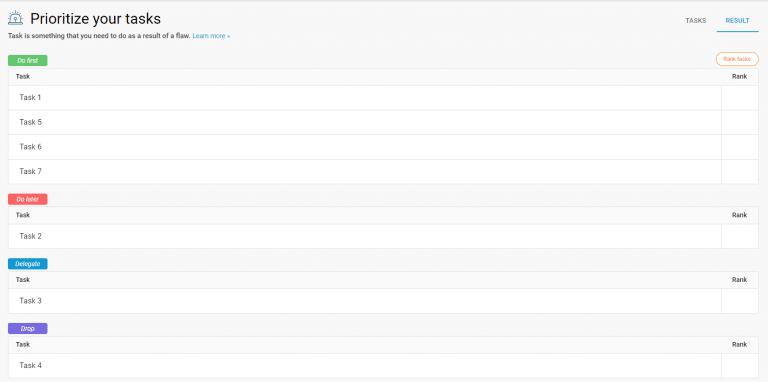A window display showcases a task prioritization tool against a gray background featuring multiple rows and columns. The top line highlights in black, "Prioritize Your Task," with subsequent lines explaining the nature and necessity of each task, particularly emphasizing tasks required due to identified flaws.

The interface uses color coding to indicate different statuses or actions associated with tasks:
- *Blue*: "Learn More" 
- *Green*: "Do First"
- *Red*: Related to coding
- *Purple*: General tasks

There are four rows labeled as Task 1, Task 5, Task 6, and Task 7, alongside a column denoting the rank of each task (1, 2, 3, 4). Each line item conveys detailed information about the task including its necessity and status, aiding in the process of prioritization. The content of tasks appears organized within tables, making it easy to comprehend and manage.

Overall, the display serves as a comprehensive visual aid for users to effectively manage their tasks by prioritizing based on their significance and immediacy.